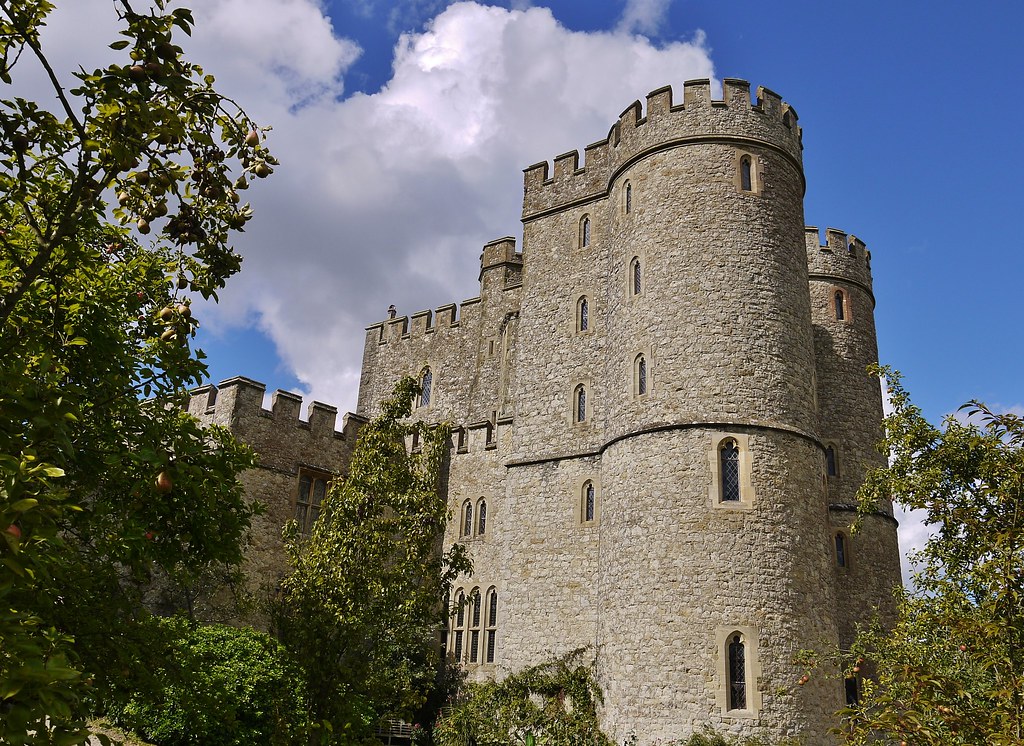The photograph captures a detailed view of a castle, focusing on a large, tall cylindrical tower made of tan stone that stands prominently in the center. The tower, reaching up to five or six stories high, features numerous small, thin windows that are arched at the top and equipped with window panes. The classic crenellations atop the tower further cement its identity as a medieval castle. Surrounding the castle are lush trees, particularly noticeable on the left side where some bear fruit, adding a burst of forest green to the scene. The blue sky overhead is dotted with a few white clouds, contributing a serene backdrop to the imposing structure. The combination of these natural and architectural elements creates an enchanting and picturesque image.